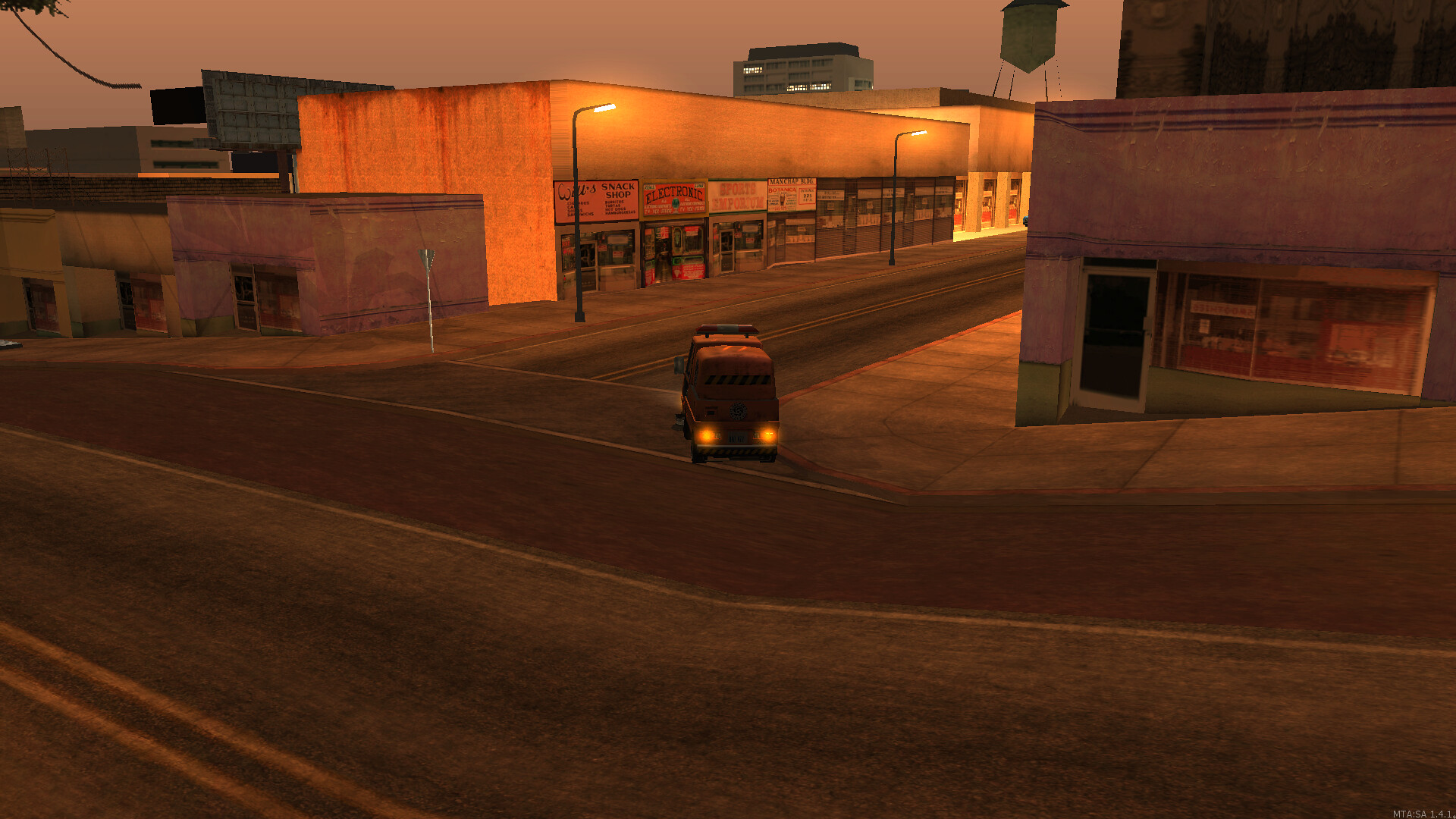The image appears to be a screenshot from a video game, likely resembling titles like GTA. The scene takes place in an urban setting at nighttime or dusk, as indicated by the dim lighting and the sky's dusky, pinkish hues suggestive of smog. Dominating the bottom part of the image is an asphalt street marked with double yellow lines on the left and a white line further right, delineating the lanes. 

On this main street, a vehicle, probably an older brown delivery or panel truck with two round yellow taillights, is turning onto a side street. To the left side of the side street, two equally spaced streetlights cast an unusual illumination on a row of doors and business signs. The buildings are largely squarish and rectangular, made of light tan concrete, and include a supermarket-like structure in the distant background. Closer to the right, there's a smaller shop with a door framed in green. Overall, the image’s graphics are clearly digital, underscoring its video game origins.